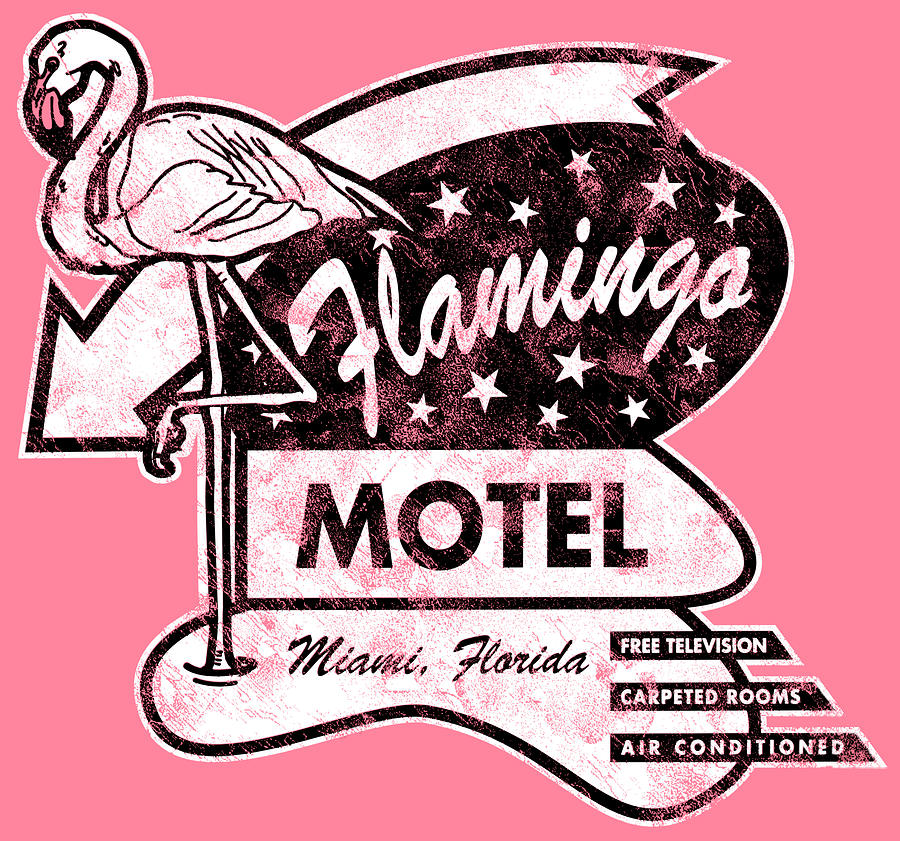This advertisement for the Flamingo Motel in Miami, Florida, features a distinct vintage aesthetic set against a flamingo pink background, aiming to capture immediate attention. Central to the design is a prominently displayed white flamingo, standing gracefully on one leg with its head bent down. Behind the flamingo, a large white arrow, outlined in black, points to the lower left, anchoring the composition with a nostalgic road sign feel.

The word "Flamingo" is elegantly written in white script within a black oval at the center of the advertisement, surrounded by white stars that add a touch of flair. Below, in a black font on a white background, the word "Motel" is prominently displayed, followed by "Miami, Florida" in a stylish black script on a similar white strip at the very bottom.

Accompanying the text, three black bars to the right detail the amenities offered, with "Free Television," "Carpeted Rooms," and "Air Conditioned" written in capitalized white letters. The entire advertisement is encased in a crisp white outline, enhancing its bold, eye-catching appearance on the pink backdrop. The overall design feels slightly distressed, adding to its retro charm and evoking a sense of nostalgic allure.